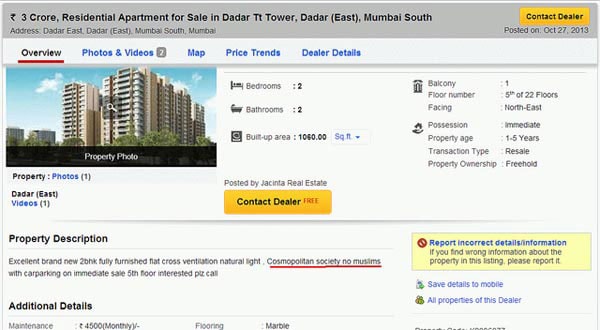For Sale: Luxury Residential Apartments in Dator Tower, Dator East, Mumbai South

Location: Dator East, Mumbai South, Mumbai

Property Details:
- Name: Dator Tower
- Type: Residential Apartments (3 core units available)
- Listing Date: October 27, 2013
- Transaction Type: Resale
- Ownership: Freehold
- Floor: 5th out of 22 floors
- Facing: Northeast
- Immediate Possession Available

Specifications:
- Built-up area: 1,060 square feet
- Bedrooms: 2
- Bathrooms: 2
- Balconies: 1

Features:
- Fully furnished
- Excellent cross-ventilation and natural light
- Carpet flooring

Amenities:
- Cosmopolitan security (no museums mentioned)

Navigation:
- Overview (current section)
- Photos & Videos: Property photos (1), Dator East videos (1)
- Map
- Price trends
- Dealer details

Contact Information:
- Yellow button to contact dealer

Additional Notes:
- Property is 1 to 5 years old
- Suitable for immediate sale
- For interested buyers, please call.